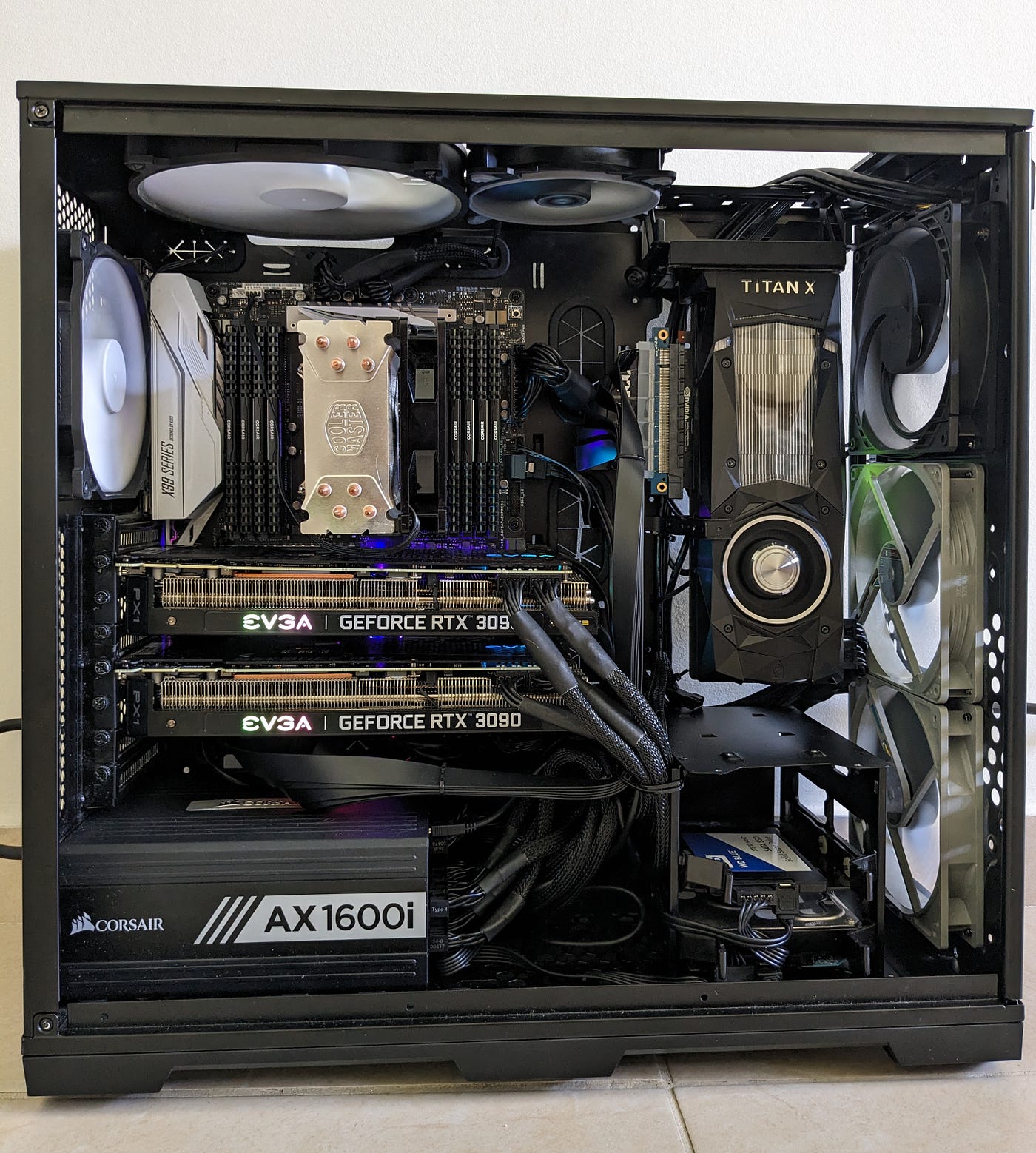This image depicts the detailed interior of a black metal computer tower, with the side case cover removed to reveal the components inside, typical of a high-performance gamer's rig. The tower sits vertically on a light gray tiled floor against a light gray wall. Dominating the view are two Nvidia GeForce RTX 3090 graphics cards from EVGA, mounted on the motherboard located on the left side. Below these cards lies a large black power supply unit from Corsair, labeled AX1600i.

The CPU is cooled by a substantial Cooler Master cooler featuring numerous copper heat pipes. Encircling the cooler, RAM modules are visible, with a total of six sticks positioned on both sides of the cooler. Towards the tower's upper section, multiple fans line the front, contributing to the overall cooling system, with additional fans mounted on the top and back of the tower.

Amidst the densely packed components, a black, white, and blue rectangular object is also visible, nestled in an open black rectangular section. Other notable components include an older Nvidia Titan X video card and various labeled sections, adding to the intricate and highly specialized setup of this computer's internal workings.